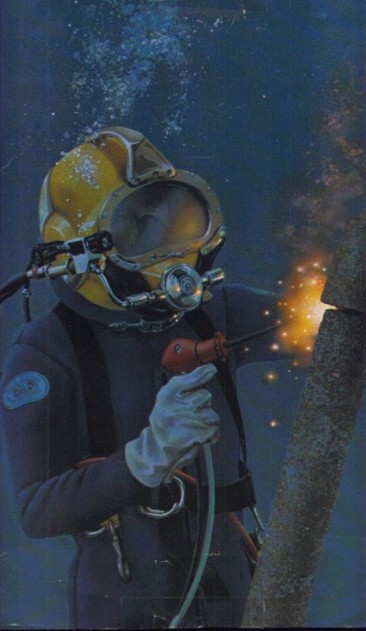This color illustration depicts a vintage underwater welding scene in vivid detail. At the forefront, an underwater welder is engaged in his task, facing right. He is clad in a gray jumpsuit with white gloves, distinguished by a blurred blue patch on his right shoulder. The welder’s gold-colored helmet, adorned with a non-illuminated black flashlight on the right side, features a face mask through which his eyes are barely visible. Immersed deep in the ocean, his surroundings are dark blue with hints of orange. The helmet emanates a cloud of bubbles, and a red welding tool in his right hand emits bright orange sparks as he repairs a rusty, angled pipe positioned in the bottom right corner of the image. The entire scene is steeped in a vintage aesthetic, giving it a timeless, historical quality.